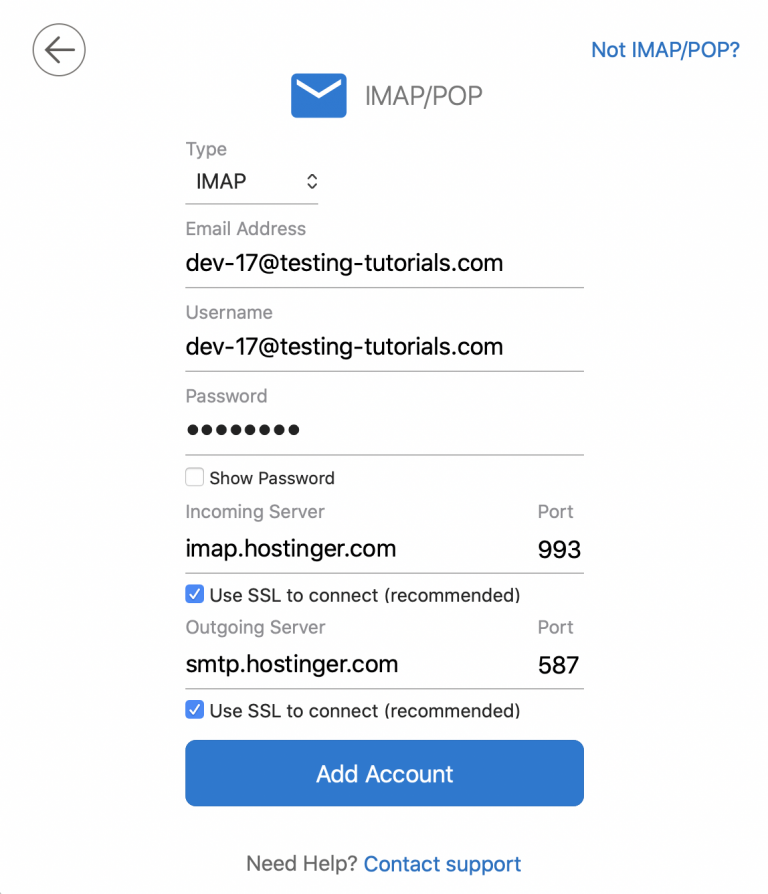The upper left corner of the image features an arrow pointing left inside a circle. To the right, there's a blue square icon resembling an envelope. Adjacent to this, it says "IMAP/POP," followed by the word "Type" and "IMAP" beneath it.

Next, the email address "DEV-17@testing-tutorials.com" is underlined. Directly below, the username "DEV-17@testing-tutorials.com" is displayed again. Following this, the word "Password" appears with eight black circles representing the masked password characters. Nearby, "Show password," along with a square checkbox, is visible.

In the next section, "Incoming server" is written in black text, followed by "imap.hostinger.com." The port number "993" is displayed in bold black text next to a small blue square with a checkmark. The words "Use SSL to connect (recommended)" appear in parentheses beside it.

Further down, "Outgoing server" is indicated, with "smtp.hostinger.com" below it, followed by the port number "587." At the bottom, inside a blue rectangle, the words "Add Account" are prominently shown.